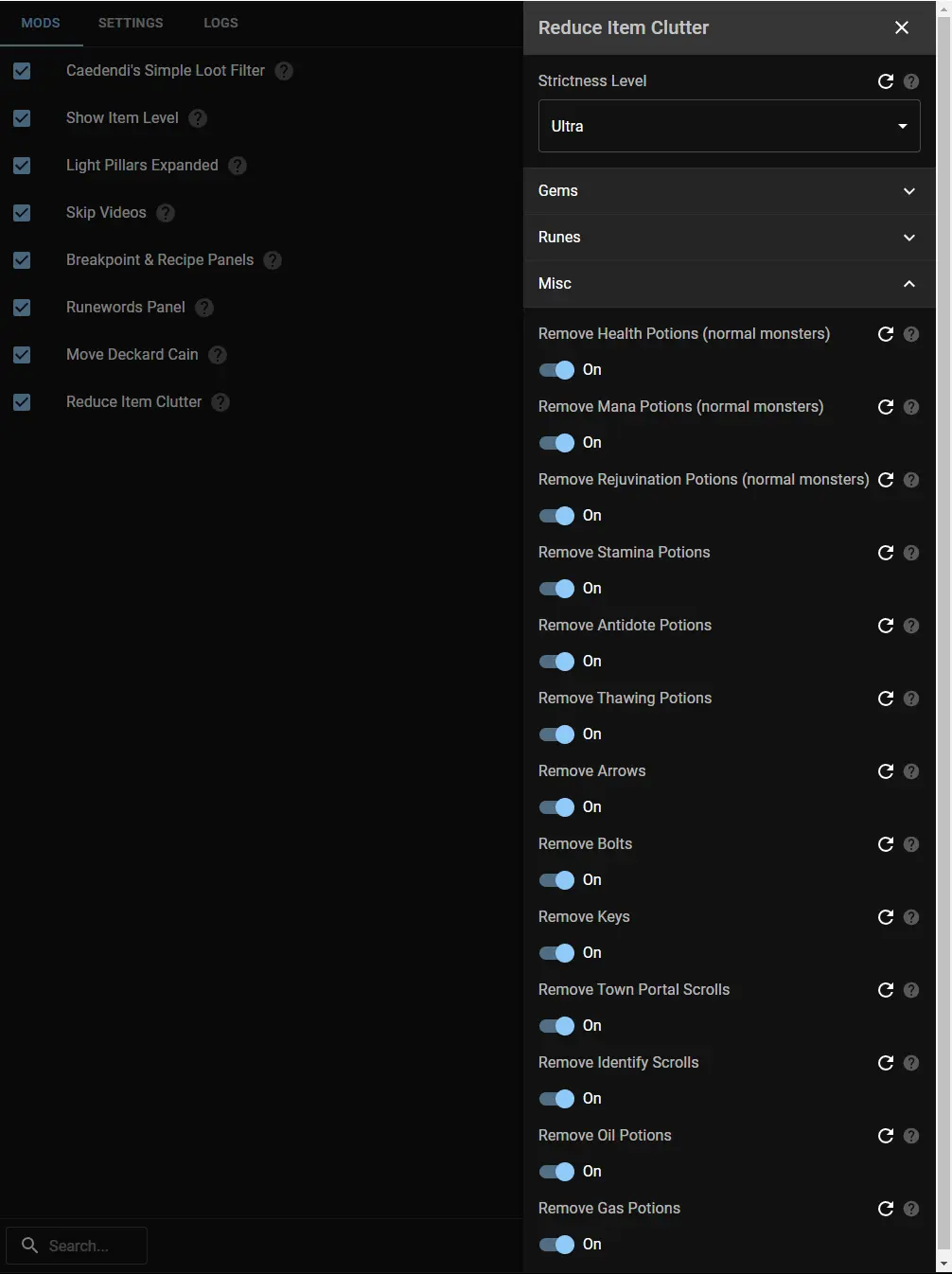This screenshot displays the settings menu within a mod for a Diablo game. The interface features a charcoal black background with "Mods," "Settings," and "Logs" listed in the upper left corner in white font. "Mods" is highlighted in blue, indicating it is the selected option.

Below, a submenu is visible, presenting various mod options in white font: "Can Dendy's Simple Loot Filter," "Show Item Level," "Light Pillars Expanded," "Skip Videos," "Breakpoint and Recipe Panels," "Rune Words Panel," "Move Deckard Cain," and "Reduce Item Clutter."

On the right side of the screen, a lighter gray rectangle showcases detailed settings for the "Reduce Item Clutter" option. It includes a dropdown menu labeled "Strictness Level" set to "Ultra," with additional categories such as "Gems," "Runes," and "Miscellaneous" that can be selected. 

Beneath these, numerous toggle options are listed, all currently enabled. These include:
- Remove Health Potions
- Remove Mana Potions
- Remove Rejuvenation Potions
- Remove Stamina Potions
- Remove Antidote Potions
- Remove Thawing Potions
- Remove Arrows
- Remove Bolts
- Remove Keys
- Remove Town Portal Scrolls

This comprehensive mod aims to streamline gameplay by minimizing item clutter in the Diablo game.